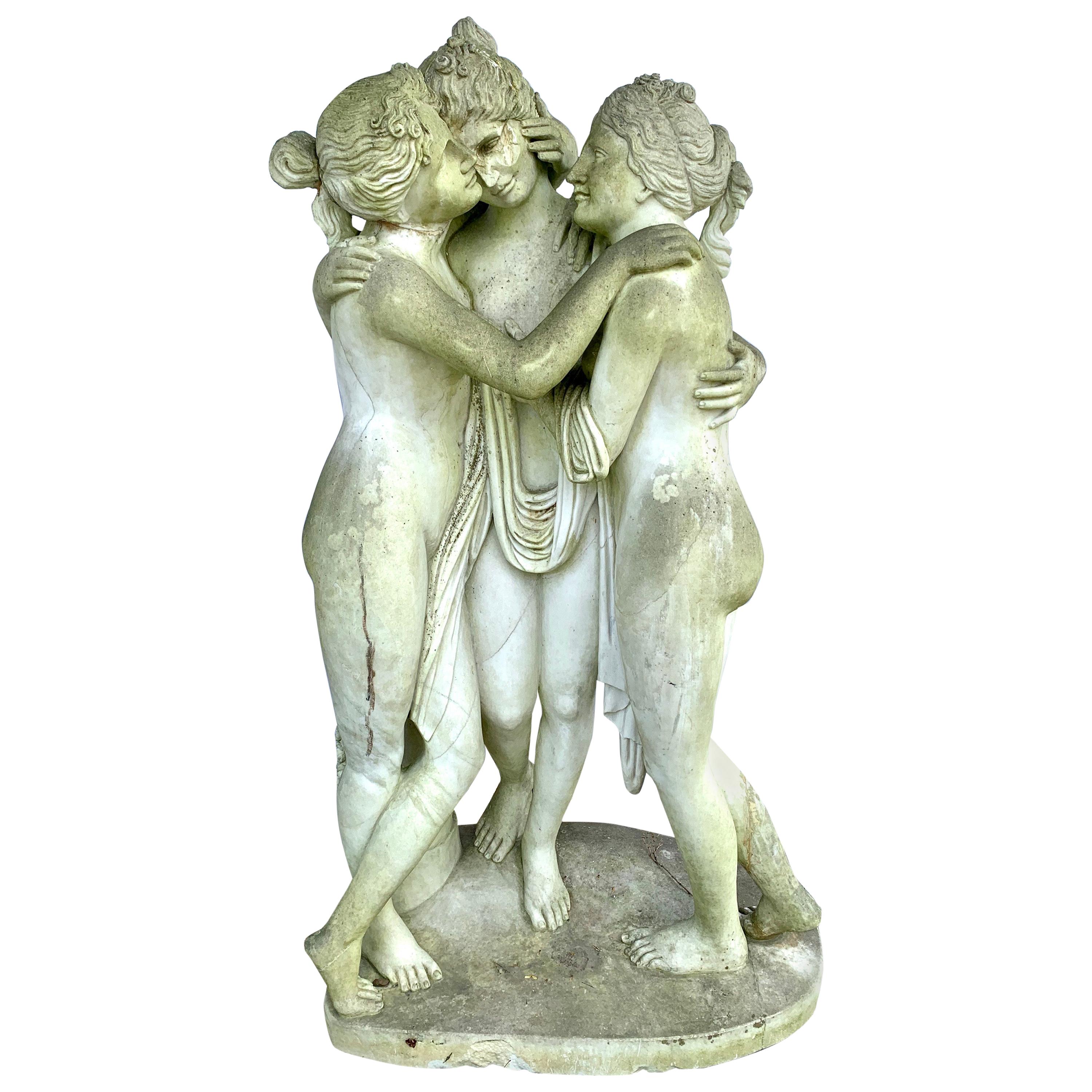This detailed depiction presents a photograph of a worn, ancient-like, marble statue, seemingly Greco-Roman, showcasing three young women standing closely together on a polished stone pedestal. Each woman, carved intricately with wavy, tied-up hair, reflects a timeless sense of age and artistry. The central figure stands facing forward with a gentle smile, tenderly resting her head on the shoulder of the woman to her right, who has one arm around her back and the other on the shoulder of the woman to her left. The middle woman's gesture encapsulates them in an intimate embrace, symbolizing deep companionship or sorrow. The woman to the left gazes downward, shrouded in the same flowing white fabric that seamlessly obscures their bodies, modestly ensuring no private areas are revealed. Opposite, the third woman, on the right, looks across with about a head’s worth of space between them. Despite slight wear and feathering on parts of the statue, the bright marble retains its enchanting elegance, illustrating a moment of shared tenderness frozen in time.